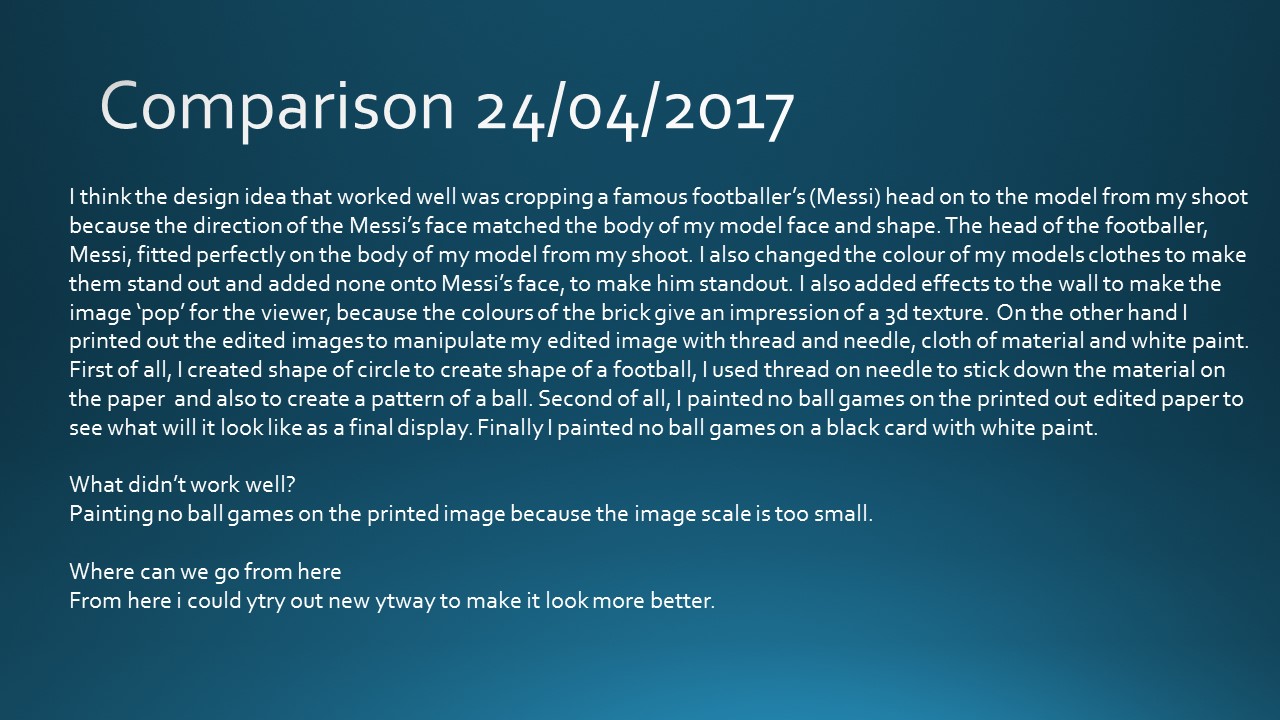The image features a blue background with white text that reads "Comparison 24/04/2017." The text includes a detailed discussion of a design project where Messi's head was cropped and placed onto a model from a photoshoot. This combination worked well because the direction and shape of Messi's face matched the model's body seamlessly. To enhance the effect, the color of the model's clothes was altered to make them stand out, while effects were added to the wall to create a vibrant and textured appearance. The colors of the bricks contribute to a 3D illusion, adding depth to the image.

Additionally, the designer used various materials and techniques to further manipulate the image. They created a circle shape to simulate a football and used thread and needle to attach material onto paper, creating a ball pattern. This was followed by painting the phrase "No ball games" on a printed edited image, despite the small scale making it less effective. Finally, "No ball games" was painted on black card with white paint as an alternative.

The final section reflects on what did not work well, particularly the issue with the scale of the painted text on the printed image, and suggests trying new methods to improve the design.